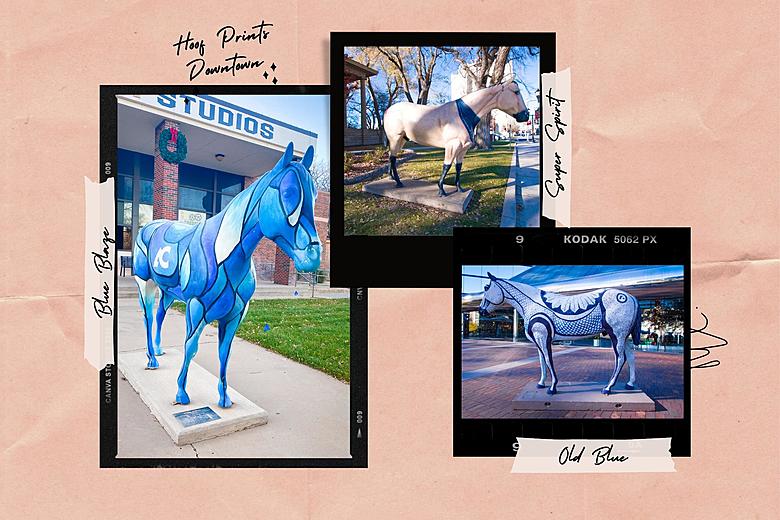The image is an advertisement styled like a scrapbook, featuring a light pink backdrop with photos that resemble Polaroid pictures. These photos are taped at the sides with masking tape, on which cursive writing is visible. The setting includes three horse sculptures. The first photograph, located on the left, shows a horse labeled "Blue Blaze" with a diamond pattern comprised of various shades of blue. The second photo, at the top, depicts a Palomino horse named "Super Spirit," notable for its cream-colored body, black legs, and feet, and an adornment of a bandana. The third image, in the bottom right corner, features "Old Blue," a sculpture adorned with a colonial-style pattern of white and blue, with a distinctive flower on its back. Each horse appears to be positioned in a downtown area, adding to the unique, vibrant, and artistic representation of the sculptures.